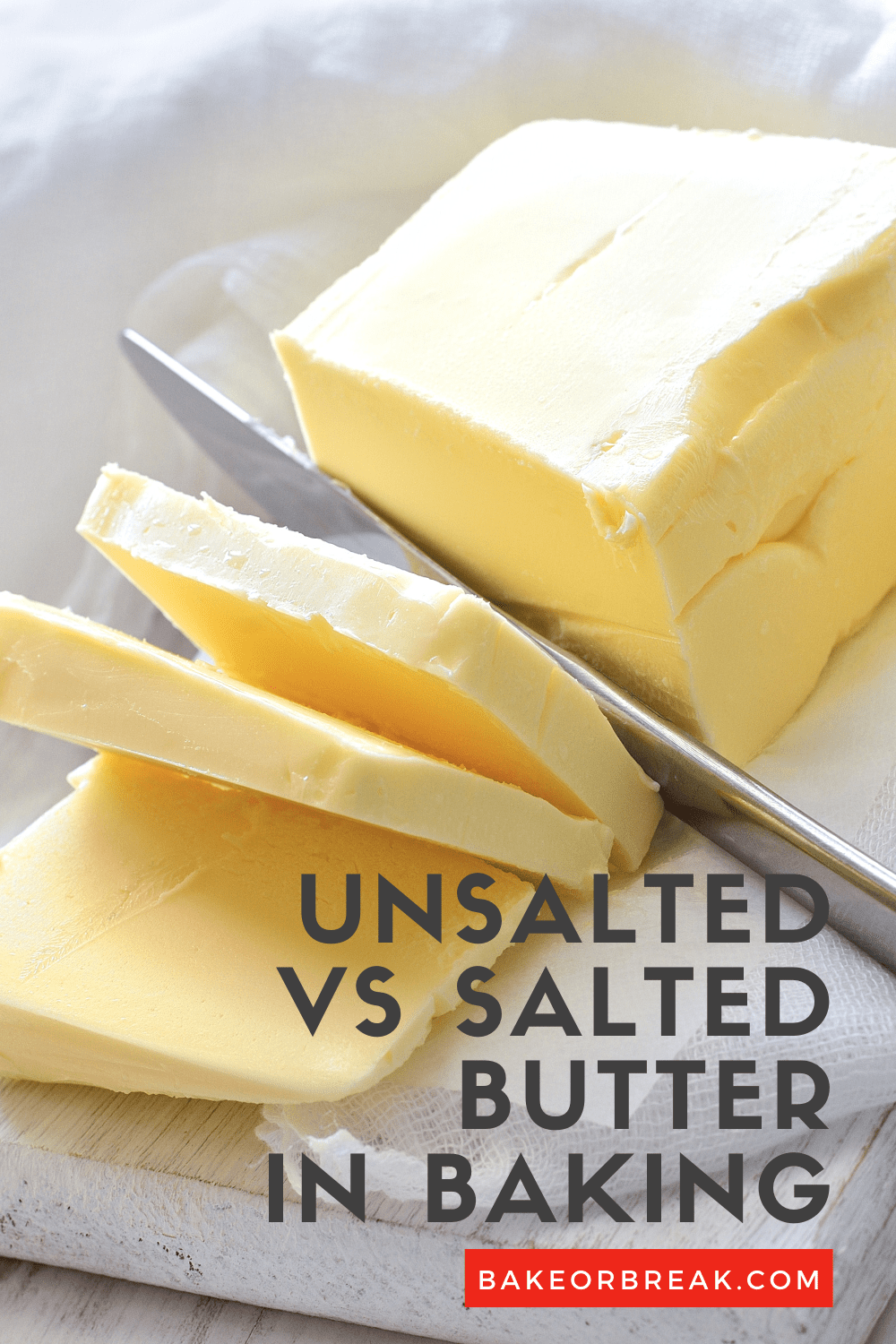The image is a close-up of a light yellow stick of butter placed on a white wooden cutting board with a piece of white cheesecloth underneath. A silver butter knife is slicing through the butter, with three slices already cut and beginning to fall. The scene does not show any hands, focusing solely on the knife and butter. In the bottom corner, gray text reads "Unsalted vs. Salted Butter in Baking," and a red rectangle with white letters says "bakeorbreak.com." The background features a crumpled white cheesecloth, adding to the rustic aesthetic of the setup.